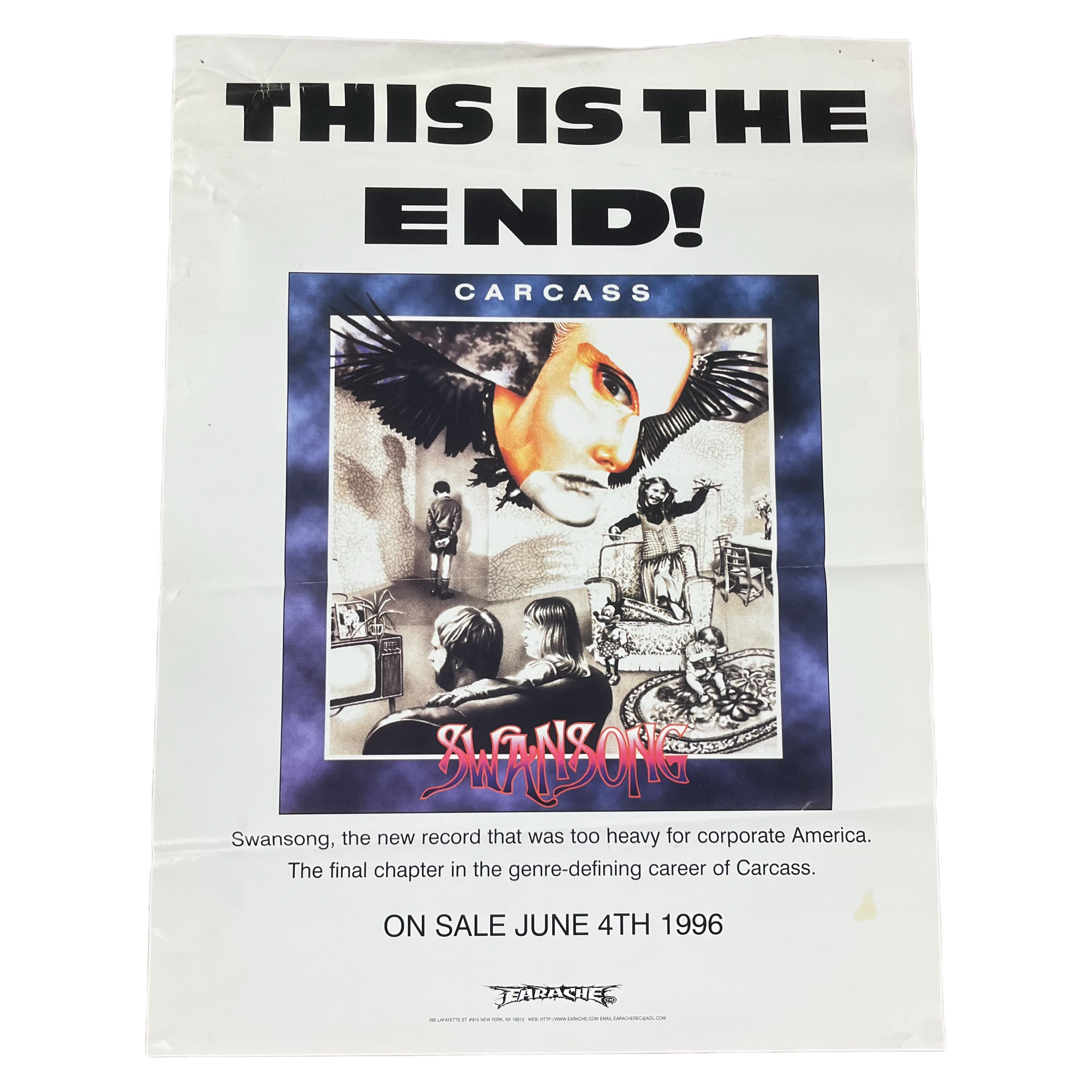This image is a detailed flyer for the band Carcass, promoting their album "Swan Song," which was released on June 4, 1996. The flyer features a stark white background with bold black capital letters at the top proclaiming, "THIS IS THE END!" In the center of the flyer is a prominent square bordered by a thick blue line, inside of which is a hand-drawn image depicting various family members—two adults sitting in front of a TV with a baby on the floor and a boy in the corner, all overshadowed by an ominous face descending from the ceiling. Above this square, the band's name "Carcass" is displayed in white capital letters, while the album title "Swan Song" appears at the bottom in vibrant pink and purple capital letters. Beneath the image, the text reads: "Swan Song. The new record that was too heavy for corporate America. The final chapter in the genre-defining career of Carcass. On sale June 4th 1996." The flyer also features the logo for their record company, Earache, tying together this compelling and genre-defining promotional material.